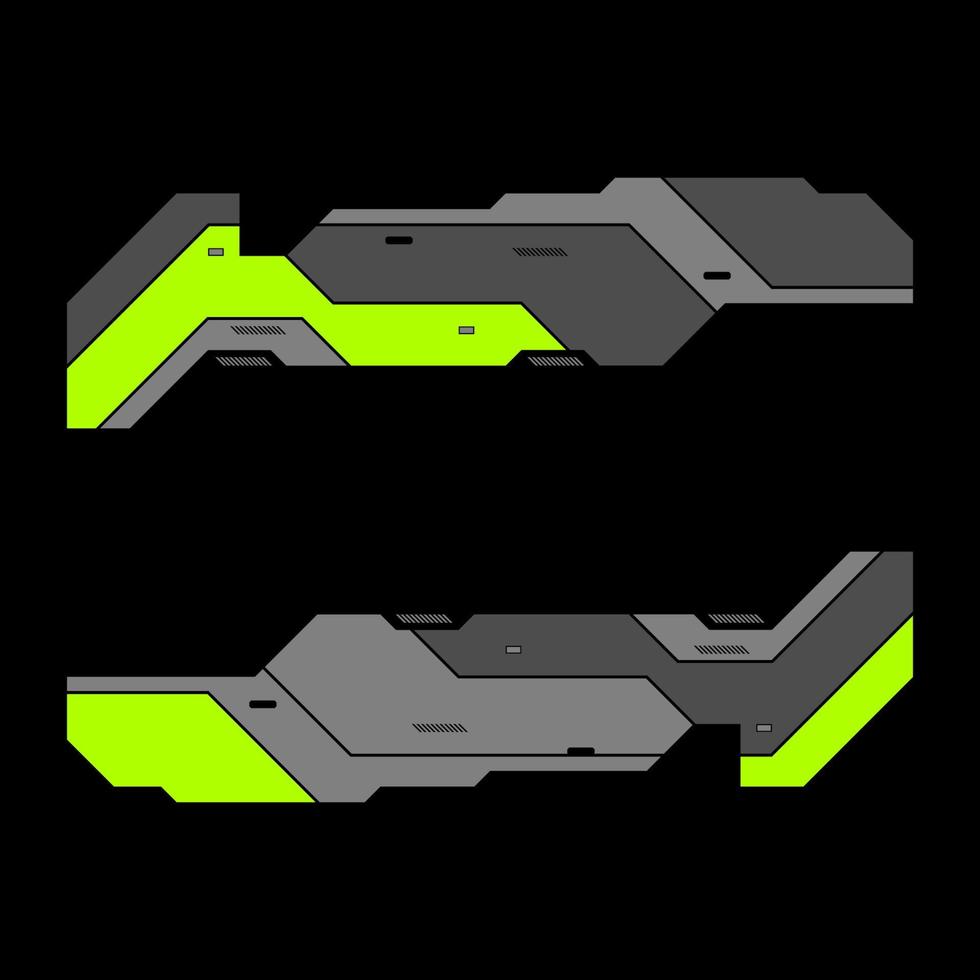The image features an intricate design pattern resembling a section of flooring. The pattern consists of interconnected lines and shapes in yellow, black, and gray tones set against a black background. The design elements are neatly arranged, with a visible space between the two main shapes, creating a balanced yet complex composition. Subtle numerical markings or details are present, adding a sense of technical specificity. The overall appearance of the design gives off a sleek, modern aesthetic, reminiscent of a 3D weapon skin in a video game, combining artistry with a sense of engineered precision.